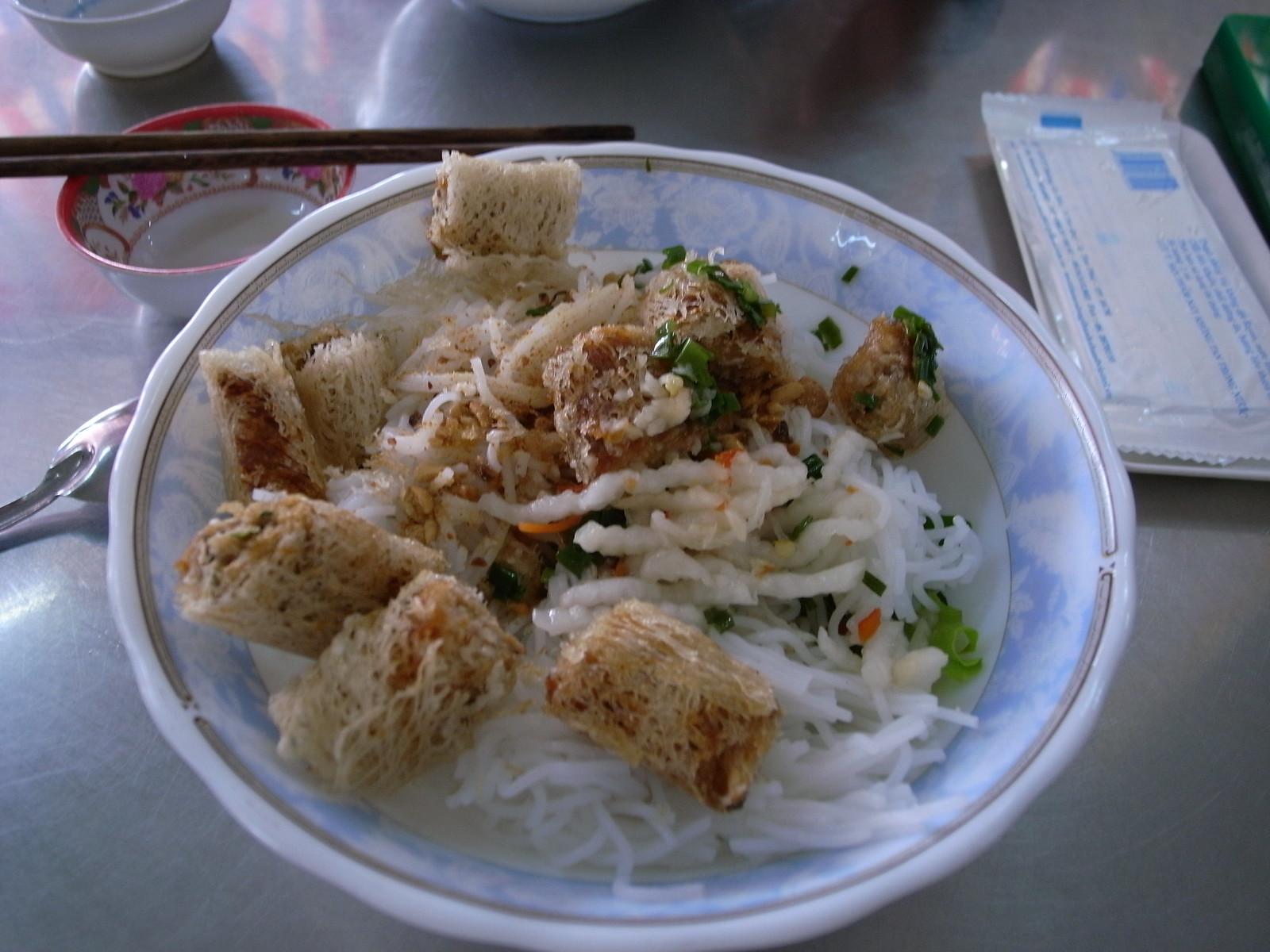This photograph showcases an Asian-inspired meal placed on a silvery-white table. At the center is a white plate filled with rice noodles, mixed with fresh vegetables such as green lettuce and possibly shredded carrots. Atop the noodles rests an assortment of small, fried dumpling-like items, which appear to be filled with vegetables. To the right of the plate is a bowl without any sauce, distinguished by brown chopsticks placed over it and a spoon positioned to its left. To the upper left of the table setting, there is a plastic container likely holding wet napkins, marked by a white wrapper with blue text. This detailed arrangement presents a visually appealing and organized meal setup.